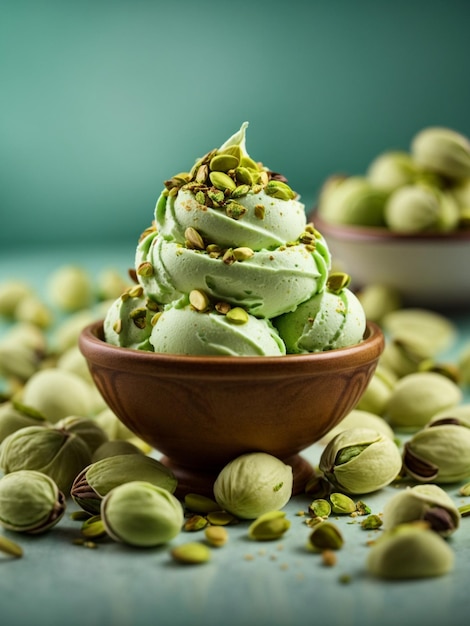The photograph features a small, shiny brown clay bowl adorned with intricate brown designs. Inside the bowl, there are three round scoops of vibrant green pistachio ice cream, topped with two layers of fat, swirled icing. The ice cream is generously sprinkled with crumbled green pistachio nuts. Surrounding the bowl on a flat, reflective blue surface are several uncracked pistachios, showcasing their distinctive green and tan shells, as well as scattered pistachio crumbs. The background consists of a blue-painted wall, adding a cool contrast to the scene, and a second bowl—white with a brown rim—filled with more pistachio nuts. The focus of the image is predominantly on the pistachio ice cream in the foreground, with the background slightly blurred to emphasize the creamy dessert and its accompanying garnishes.